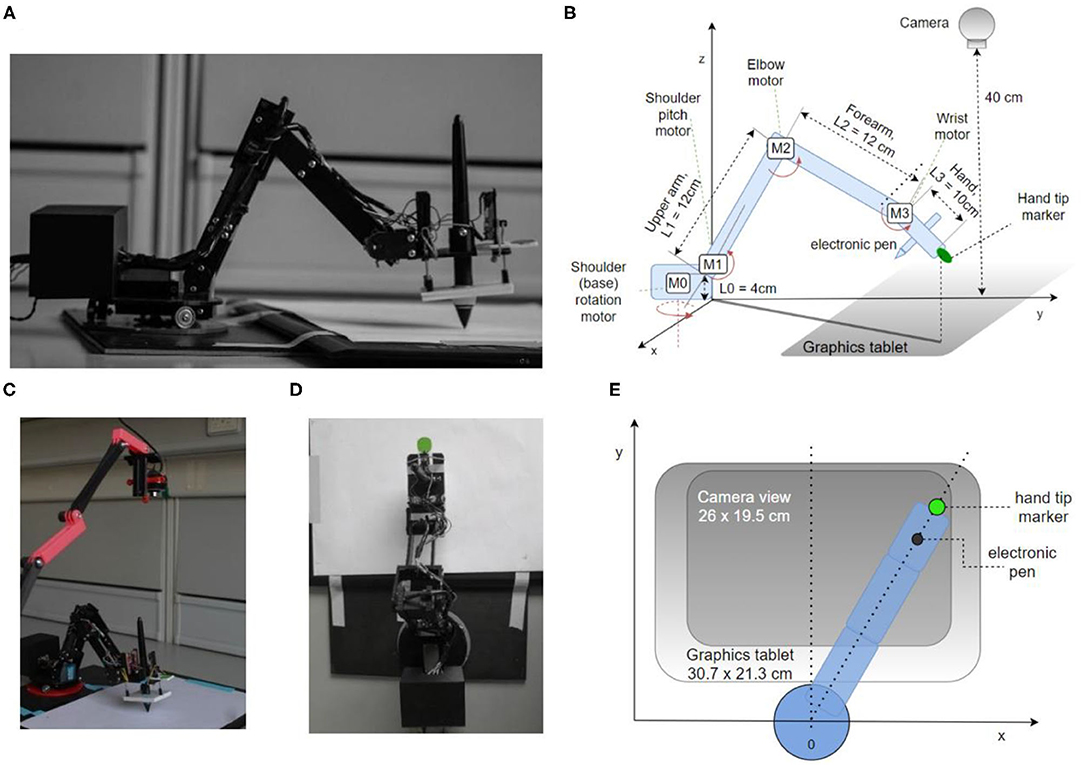The image comprises five labeled sub-images (A-E) illustrating various perspectives and diagrams of a black robotic hand engaged in drawing on a piece of paper laid on a black graphics tablet. In Image A, a side view showcases the entire robotic hand holding a stylus or pen, actively drawing. Image B presents a detailed diagram with measurements and labels for each component, including the shoulder base, various motors, upper arm, forearm, wrist, and the electronic pen. The diagram clarifies the dimensions and spatial orientation using X, Y, and Z axes. Image C offers a top view of the robotic hand, highlighting its position relative to the graphics tablet and an additional robotic arm positioned above. Image D mirrors this top-down perspective, specifically pointing out a green spot on the paper. Lastly, Image E delivers another top-down diagram emphasizing the spatial layout of the robotic hand and its interaction with the graphics tablet, reiterating key labels and measurements from Image B. Overall, the presentation integrates multiple viewpoints and technical specifications, illustrating the intricacies of the robotic hand and its functionality.